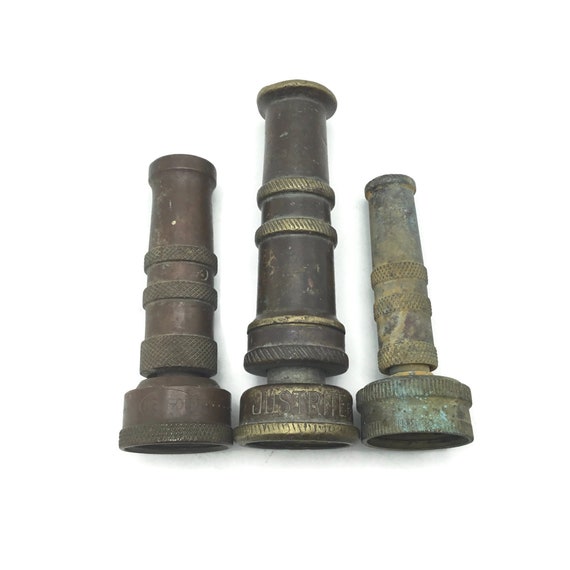The photograph features three metal garden hose nozzles, each showcasing signs of wear from usage. On the left, the first nozzle, notable for its almost brown hue, features three grip-textured lines for ease of handling, and the bottom section where it attaches to the hose is prominently visible. The middle nozzle, the longest of the trio, displays two grip lines and has a stamped inscription near the attachment point, potentially identifying the brand, though the text is not entirely legible. The third nozzle on the far right appears the most worn and possibly dirty. It shares similarities with the first nozzle, having three grip lines—two near the top and one near the bottom—yet it is thinner and smaller in size.